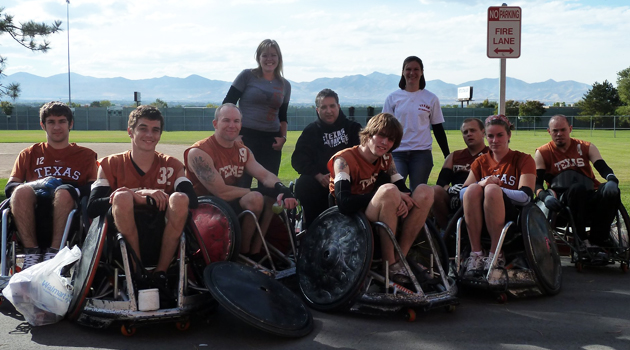A group of ten athletes, prominently clad in burnt orange shirts with the word "Texas" and varying numbers, gather outside for a team photo. Eight of them sit in specialized sport wheelchairs with large, tilted wheels, suggesting they are adapted for their sport. Among these, one athlete, a woman, stands out with blue sleeves on her forearms. In contrast, two women, likely coaches, stand behind the seated athletes—one in a gray shirt with black sleeves, a big smile, and black pants, and the other in a simple white shirt with blue jeans. A man in a black sweatshirt with "Texas" is either sitting or stooping between them. Behind this group, a backdrop of mountains, clouds, and a chain-link fence with trees is visible. A conspicuous "No Parking, Fire Lane" sign with double arrows stands out above the scene, adding context to their location near a parking lot.